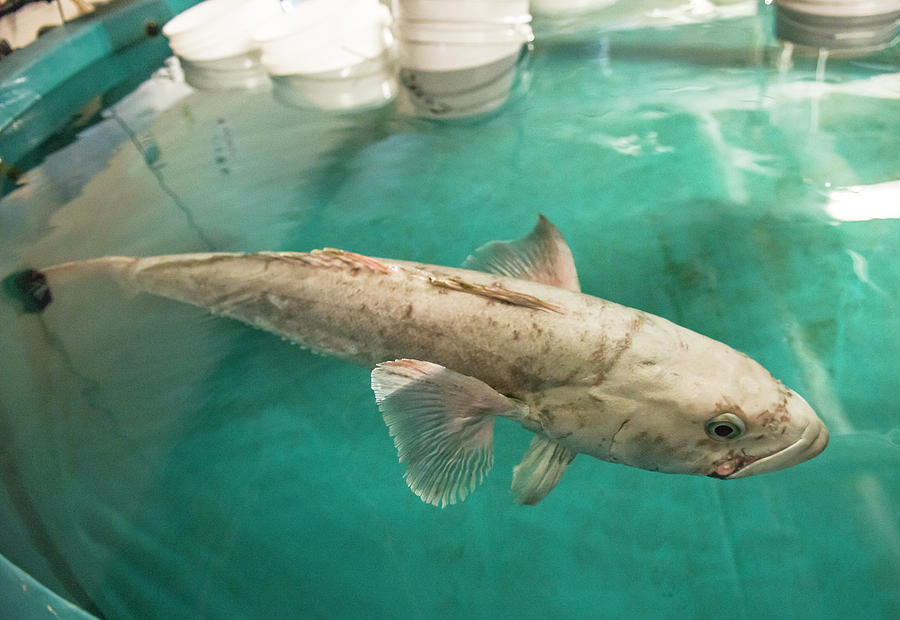This image captures a detailed close-up of a pale, elongated fish—likely a koi—swimming in a man-made pool or tank with a teal-blue hue. The fish, almost completely white with dark gray specks and hints of green and brown on its body, has distinctive black eyes edged with a light bluish-white hue. It exhibits multiple fins: two side fins, a bottom dorsal fin, and a top fin, along with a tail and possibly some spiky features. 

In the background, several white plastic buckets float, slightly blurred within the water. The surrounding pool structure has walls that appear off-white and slightly dirty above water but cleaner and more polished below the surface. The pool's edge features a deep bluish-green tone, reflecting the lighting, likely a mix of natural light and artificial illumination. The overall scene has an aquatic ambiance suggestive of either a fish breeding facility or an aquarium setting.